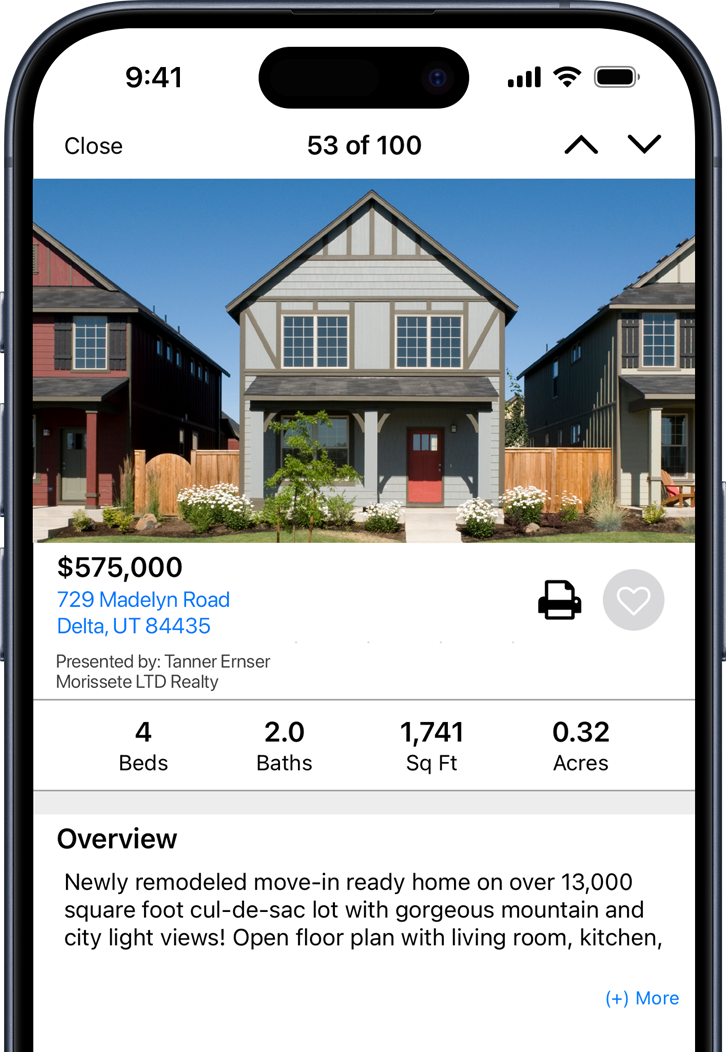In the center of the image, there is a close-up of an iPhone, with its power button visible on the top right edge and volume buttons prominently on the left side edge. The top part of the image showcases the black camera of the iPhone. Below the camera, there is a light blue rectangular box with white text that reads "Residential." Above this box, the white text indicates the time as "10:10 p.m." To the right, a battery icon shows it is fully charged, and next to it, the text "100%" is displayed.

To the left of "Residential," a white arrow and the word "Back" are visible. Underneath this, a transparent black rectangular box contains white text on the left side that reads "Showing 20 of 44."

Centered in the mid-section of the screen is an image of a light gray and beige house with a slightly tall wooden fence on either side. The bright blue sky forms the background. Adjacent houses are partially visible on each side of the main house image.

Another image of a house is shown beneath this. The second house is similar in color, light gray and beige, with a dark gray roof. At the bottom left of each house image, the price of the house is displayed. For instance, the first house is priced at "$250,000." Below the price, the address is listed, and to the right, details about the house are provided, such as "three beds, three baths, and 1,220 square feet." Similarly, the second house's price is noted as "$250,000," with its details reading "three beds, 2.5 baths, and 1,120 square feet."